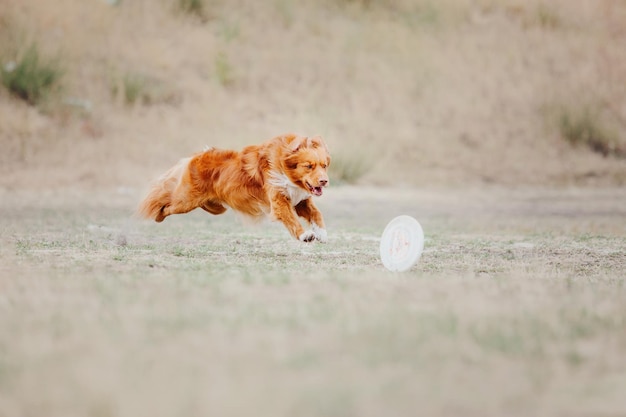This outdoor photograph captures a lively scene, featuring a dog energetically chasing a white frisbee across a low-cut grassy field on a clear day. The background and foreground are intentionally blurred, drawing focus to the midsection of the image where the action unfolds. The dog, possibly a young collie or a golden retriever with shaggy brown fur and a white chest, is captured mid-leap with all paws off the ground, running from left to right. The dog’s intent gaze and slightly open mouth highlight its determination to catch the frisbee, which rolls on its edge away from him. The grass, mostly dead-looking with occasional green patches, frames the dynamic motion of the central scene. The entire photograph emphasizes the joy and vigor of the dog in pursuit, with no other distractions in the frame.